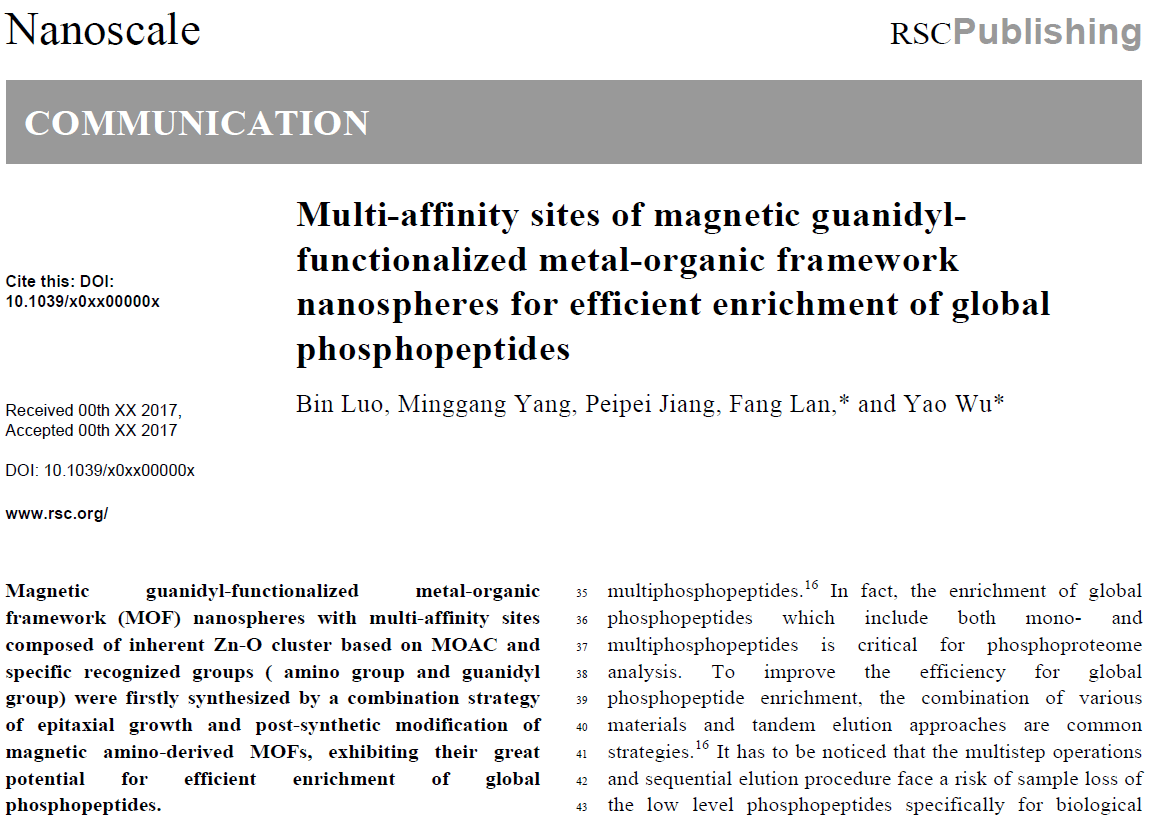**Descriptive Caption:**

At the top, the image showcases the title "Nanoscale RCS Publishing" in a gray rectangular box labeled "Communication." Below, the headline reads: "Multi-Affinity Sites of Magnetic Guanidyl Functionalized Metal-Organic Framework Nanospheres for Efficient Enrichment of Global Phosphopeptides."

The main body of the text describes a study on magnetic guanidyl-functionalized metal-organic framework (MOF) nanospheres, highlighting their advanced features. These MOF nanospheres possess multi-affinity sites, with inherent ZnO clusters forming the core of the MOF. They are further enhanced with specific recognition groups, including amino and guanidyl groups. This novel synthesis is achieved through a combination strategy involving the exataxel group and post-synthetic modification of magnetic amino-derived MOFs.

The image emphasizes the significant potential of these MOF nanospheres, particularly in the efficient enrichment of global phosphopeptides. Enrichment includes both mono- and multi-phosphopeptides, which is critical for comprehensive phosphoproteome analysis.